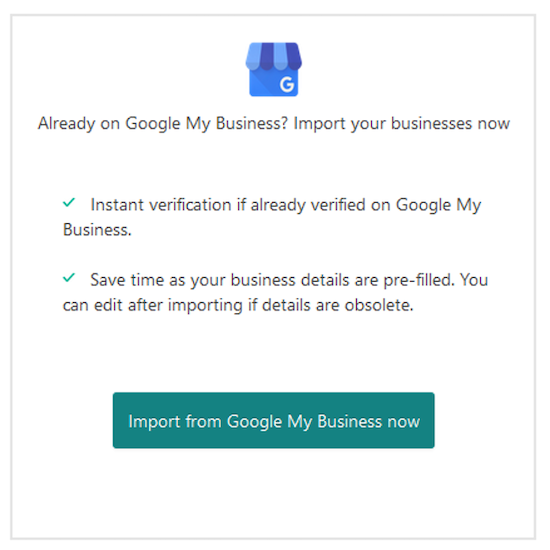The site is framed by a shaded light gray outline, forming a large box with a white center. At the top center of the white space, there's a blue square featuring a white "G" in the corner. The square is topped with an awning that resembles a small store's canopy, colored in light blue and navy.

Beneath this blue square, the text "Already on Google My Business?" is written in black, followed by the prompt "Import your businesses now." Below this, additional text is spaced out clearly:
- "Instant verification if already verified on Google My Business," accompanied by a small green check mark.
- "Save time as your business details are prefilled. You can edit after importing if details are obsolete," also marked with a green check mark.

In the middle of the page, a green banner stretches horizontally, displaying the message "Import from Google My Business now" in white text, indicating it's a clickable button. 

The bottom of the page mirrors the site's gray outline, enclosing the white spaces on either side and the top and bottom.